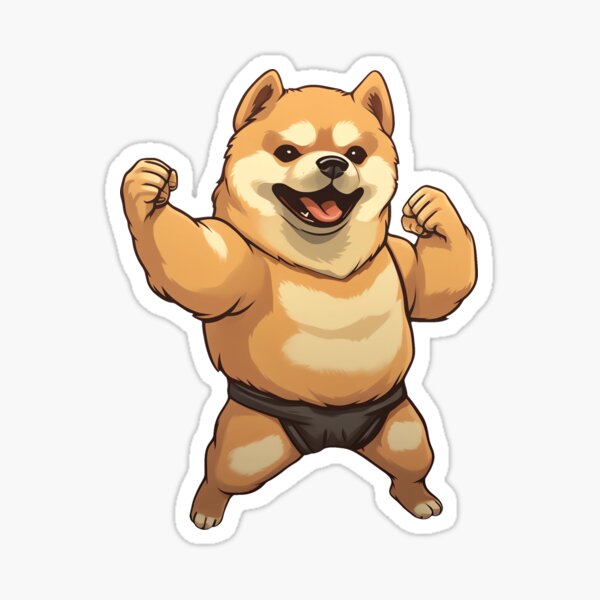The image is a rectangular, vertically oriented artwork with an off-white background. At the center, there's an embossed, cartoonish depiction of a muscular dog resembling a Shiba Inu, the mascot for a cryptocurrency. The dog, standing upright on its hind legs as if human, is poised in a boxing stance with clenched fists. Its body is notably buff, showcasing well-defined muscles. The canine is light brown with lighter beige or creamy markings, particularly around its mouth, eyes, chest, and knee areas. It features expressive black eyes, a black nose, and an open mouth revealing a red tongue, giving it a happy demeanor. The dog is dressed in dark-colored shorts reminiscent of sumo wrestler attire. This central motif is outlined with a white border, enhancing its sticker-like appearance against the solid backdrop.